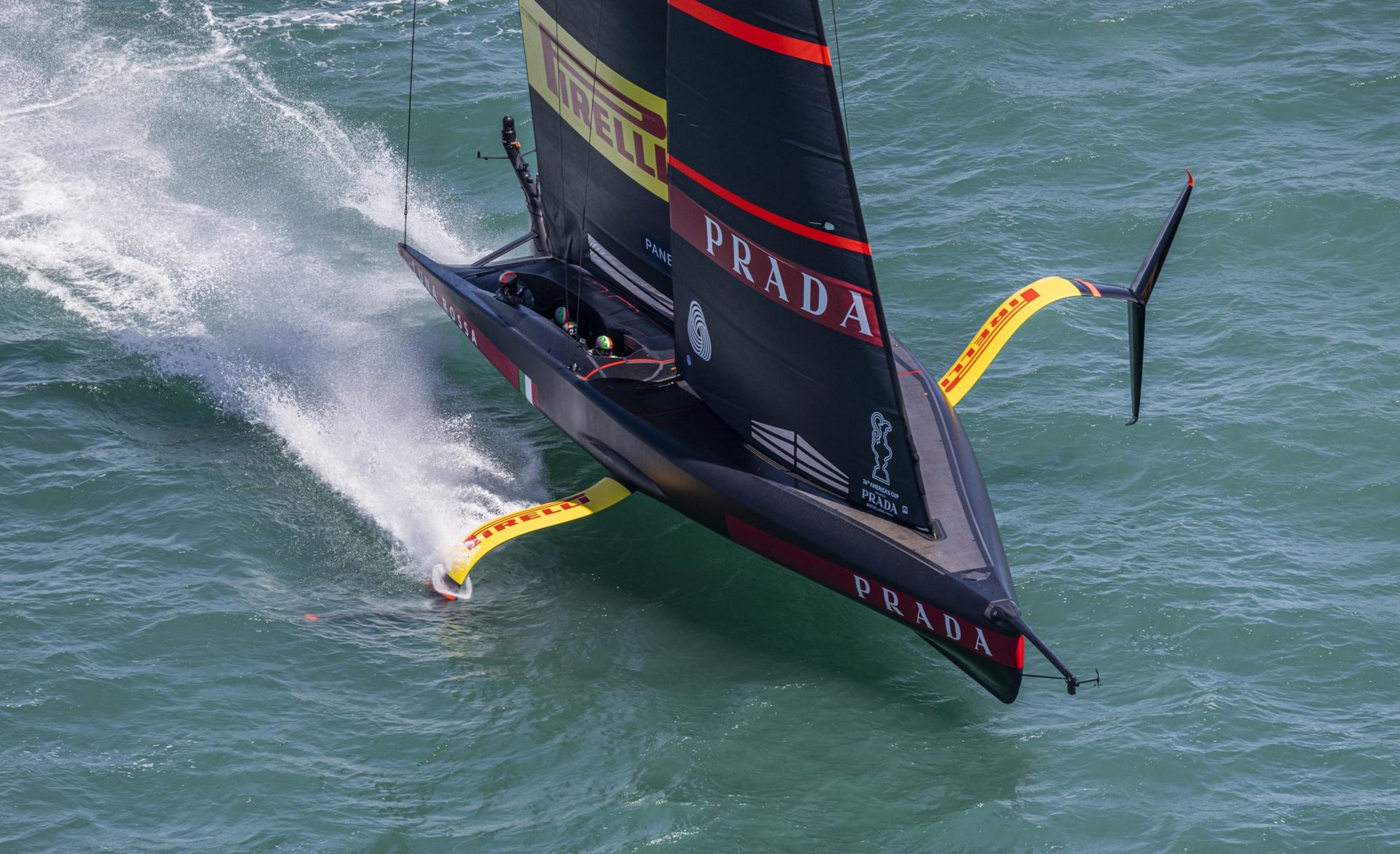This is an aerial color photograph of a sleek, high-speed racing sailboat on the ocean, prominently branded with "Prada" and "Pirelli" logos. The boat itself is an elegant black with a distinctive red stripe down the middle, featuring the name "Prada" in striking white letters. It has two main sails: the front sail is black with bold red stripes and bears the "Prada" logo on a red background, while the rear sail showcases a yellow banner with "Pirelli" written in red. Extending from either side of the boat are aerodynamic wings, painted in yellow and contributing to the vessel's cutting-edge design; one wing even has a black propeller-like feature. The boat is racing at high speed, creating a giant, frothy wake, seen as a white trail against the blue-green ocean water. The photograph captures the boat slightly lifted off the water, emphasizing its velocity and advanced engineering. Sailors on board are barely visible, dwarfed by the grandeur and modernity of the racing sailboat.